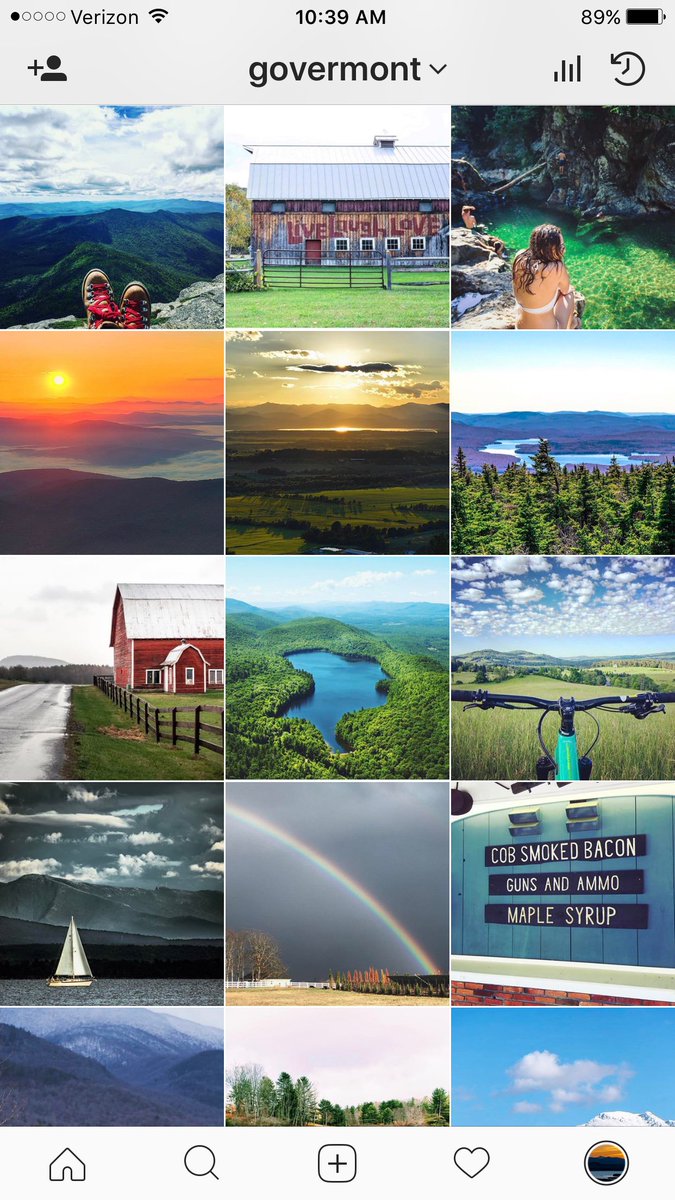Screenshot taken at 10:39 AM with Verizon showing a good signal and 89% battery. The location displayed is Govermont. The image is a collage capturing the serene beauty of the Govermont region. 

1. **Person Relaxing**: A partial view of a person reclined on the rocks, with only their shoes visible, showcasing a breathtaking overlook of the verdant mountains.
2. **Old Barn**: An old barn with the phrase "Live, Laugh, Love" painted on its side.
3. **Backyard Pool**: People in bathing suits enjoying a pool in a backyard.
4. **Sunsets**: Several stunning sunset shots over the mountains.
5. **Mountainous Landscape**: Overlooking lush green mountains with a river or lake winding through the valley.
6. **Country Road**: A picturesque country road passing by the "Live, Laugh, Love" barn.
7. **Aerial Lake**: An aerial shot of a lake resembling the shape of a lion.
8. **Electric Bike**: Handlebars of an electric bike next to a picturesque hay field.
9. **Sailboat**: A sailboat gliding on a lake, framed by distant mountains.
10. **Local Store**: A quaint local store advertising a mix of goods, including cob-smoked bacon, guns and ammo, and maple syrup, with handmade signs burnt into wood.
11. **Rainbow**: A vivid rainbow arching across the sky, adding a touch of magic to the landscape.